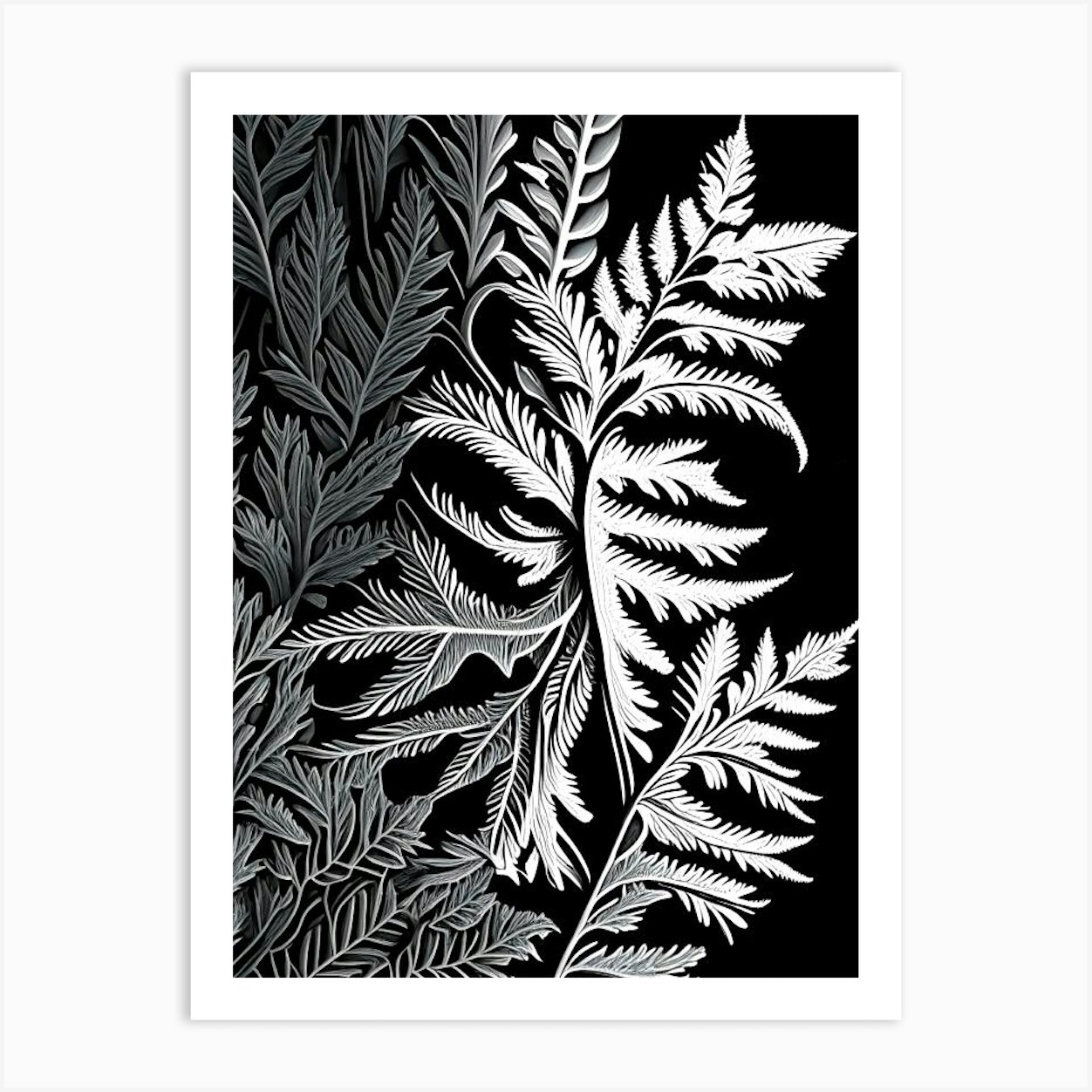The image depicts a beautiful, detailed painting framed by a white border, resembling a canvas or a white picture frame. The inner background of the painting is completely black, providing a striking contrast to the white and gray illustration of leaves and branches. The leaves appear intricately connected, and their coloration transitions from darker shades of gray on the left, hinting at possible green tones in a natural setting, to whiter shades as they extend upwards along the stems. The composition is clear, and the setting is bright, highlighting the meticulous details of the leaves and branches. There are no words or numbers present in the image, focusing solely on the elegant, monochromatic flora against the rich black backdrop.